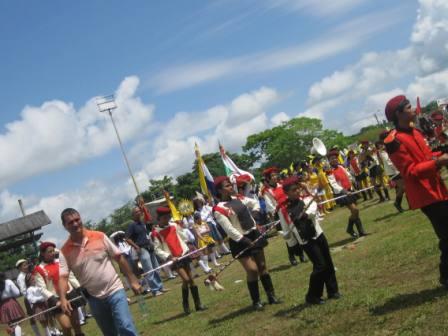In this vibrant outdoor scene, a large group of people are gathered on a grassy field, engaged in what appears to be a parade. Many participants are holding musical instruments, and there is a variety of vibrant flags on display. Some individuals are dressed in black and white uniforms, while others are in striking red and black uniforms, adding to the festive atmosphere. Several people are also seen holding batons, signifying a possible marching band or performance group. The background is adorned with lush green trees, enhancing the natural beauty of the scene. Above, the sky is a bright blue with a few scattered clouds, completing the picturesque setting of this lively event.